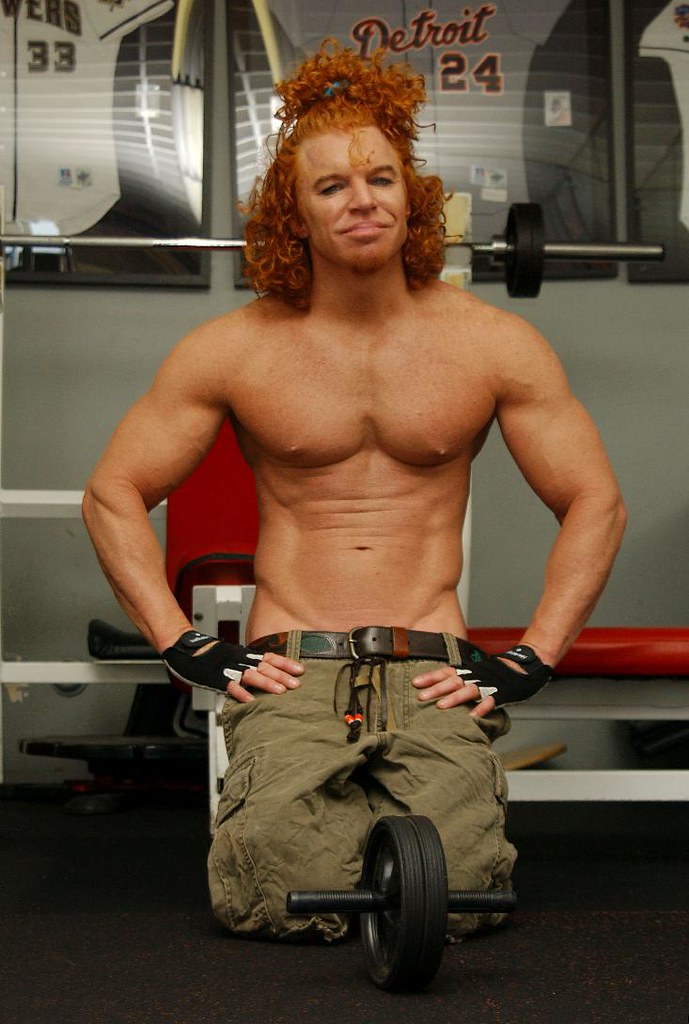The image captures the comedian Carrot Top at a gym, kneeling and facing the camera with his hands on his hips. He is shirtless, revealing his tanned, very muscular physique, including well-defined abs. Carrot Top's signature red, curly shoulder-length hair is partially pulled back into a ponytail on the top of his head. He is wearing black and white weightlifting gloves, along with army green shorts or pants secured with a black leather belt. In front of him lies an ab roller with two wheels and handles. Behind him, there is a red and white bench press machine, along with barbells and a barbell rack to his left. The gym's wall is adorned with framed baseball jerseys, most prominently featuring a gray "Detroit 24" jersey and another white jersey with the number 33.